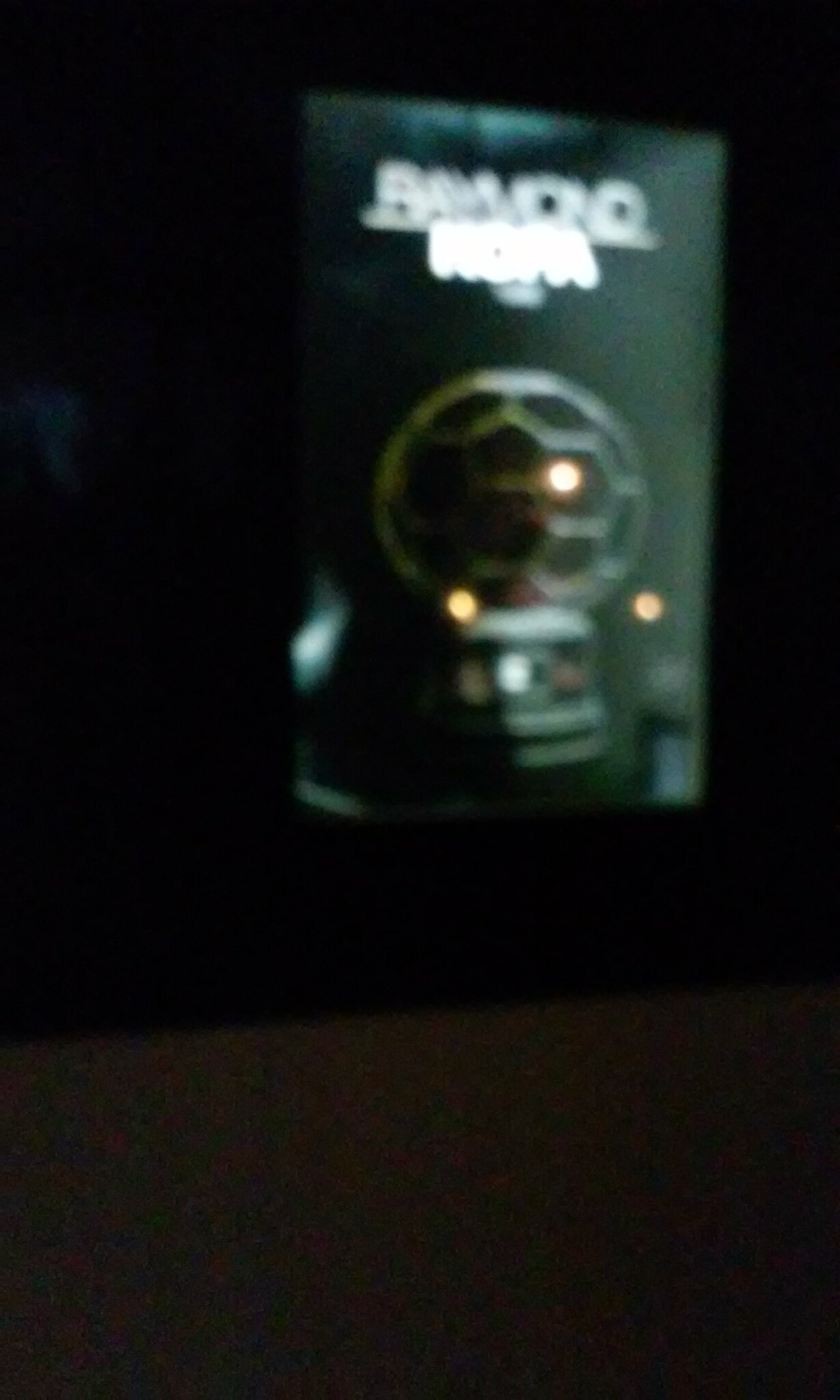The image is a close-up, albeit blurry, shot of a black package resting on the edge of a dark-colored table. Atop the package, a see-through, glass-like sphere is prominently displayed on a rounded, black base. This clear object appears small, but its exact size is indeterminable due to the lack of reference points. The package features a silver label, although the text remains unreadable due to the blurriness. The background reveals a section of what seems to be a dark brown carpet or tile floor. The overall photograph is both blurry and heavily zoomed in, making finer details difficult to discern.